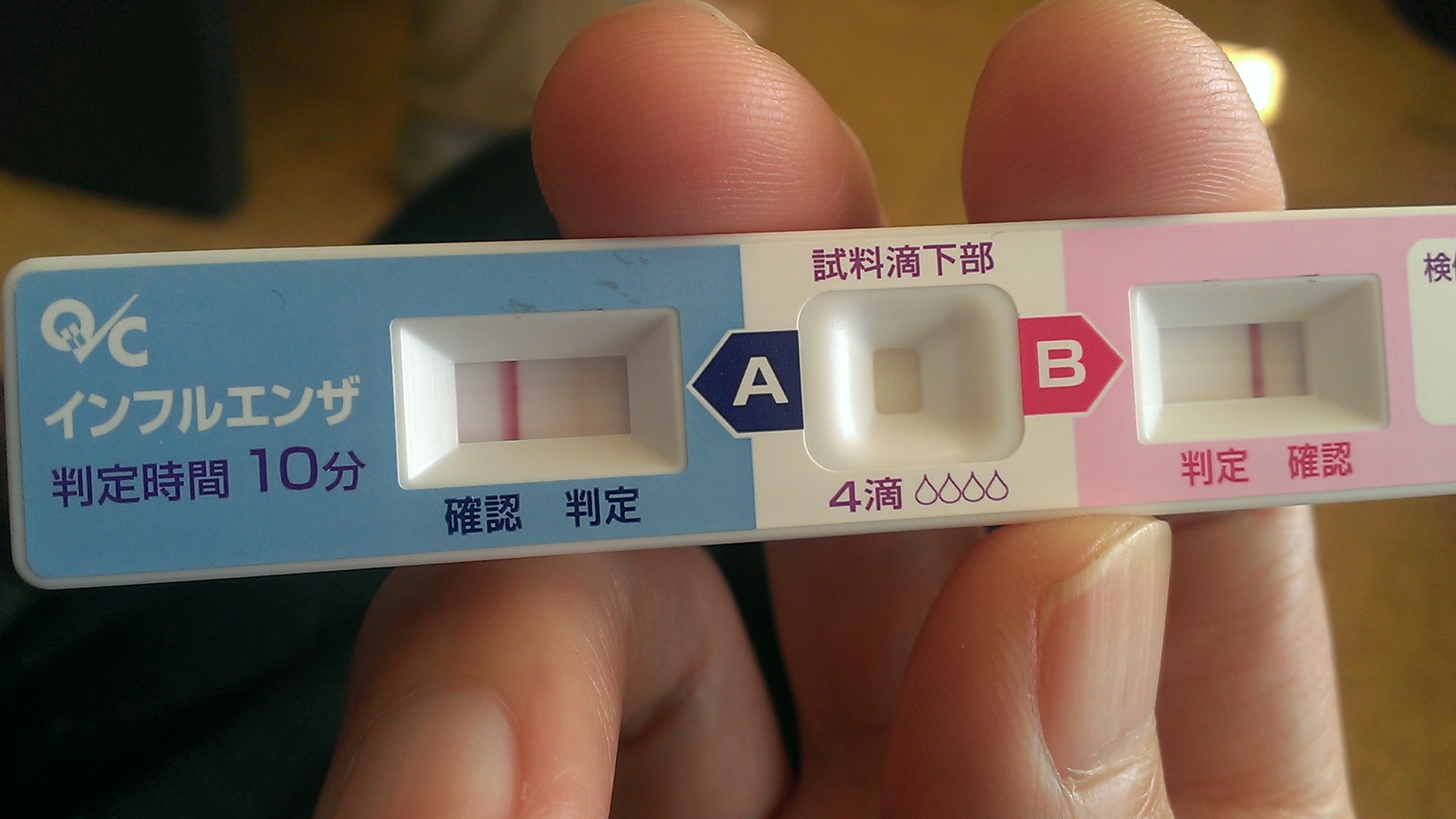A hand is prominently holding a pregnancy test in the left side of the image. The test is a colored stick, predominantly blue, featuring a white square with a pink line through it. The stick appears to have Chinese writing on it. To the right of the pregnancy test, there is another section marked with a pink option labeled 'B,' framed with a pink border, a pink line, and another white square. In between markings 'A' and 'B,' there is an area with a white border, a white square in the center, and the number '4' clearly visible. Surrounding this central area are four small icons depicting water droplets. More Chinese characters are present within the image. The background is somewhat blurred, revealing a wooden floor.